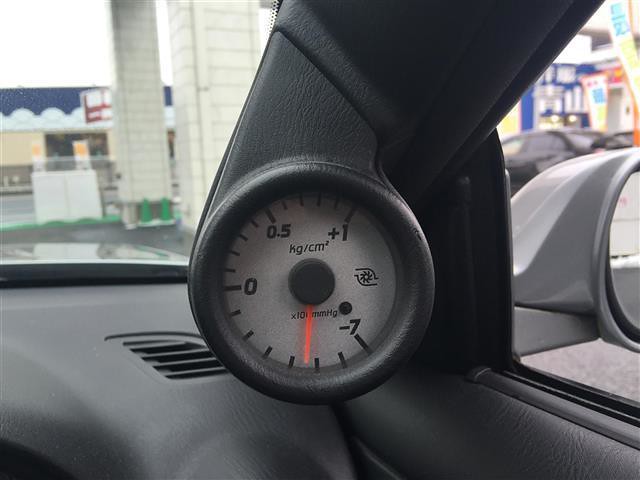This photograph, taken from the passenger seat of a vehicle, captures a scene both inside and outside of the car on what appears to be a bright, possibly overcast, day. The viewer's eyes are drawn to a unique, round gauge resembling a speedometer or altimeter, prominently mounted on the passenger side of the dash. This intriguing device has a white face with dial markings ranging from -7 to +1, with -7 positioned at the lower right and +1 at the upper right, though its purpose remains unclear.

Outside the vehicle, the scene reveals details of a gas station through the passenger window. The gas pumps, adorned with numerous numbers and signs, contribute to the bustling, everyday setting. The gray mounting of the side mirror, along with a sliver of the mirror itself, is also visible through the same window. The windshield offers a glimpse of a distant storefront, subtly anchoring the viewer in a familiar roadside environment. Overall, the image juxtaposes the mystery of the dashboard gauge against the mundane backdrop of a gas station, creating an intriguing and detailed frame.